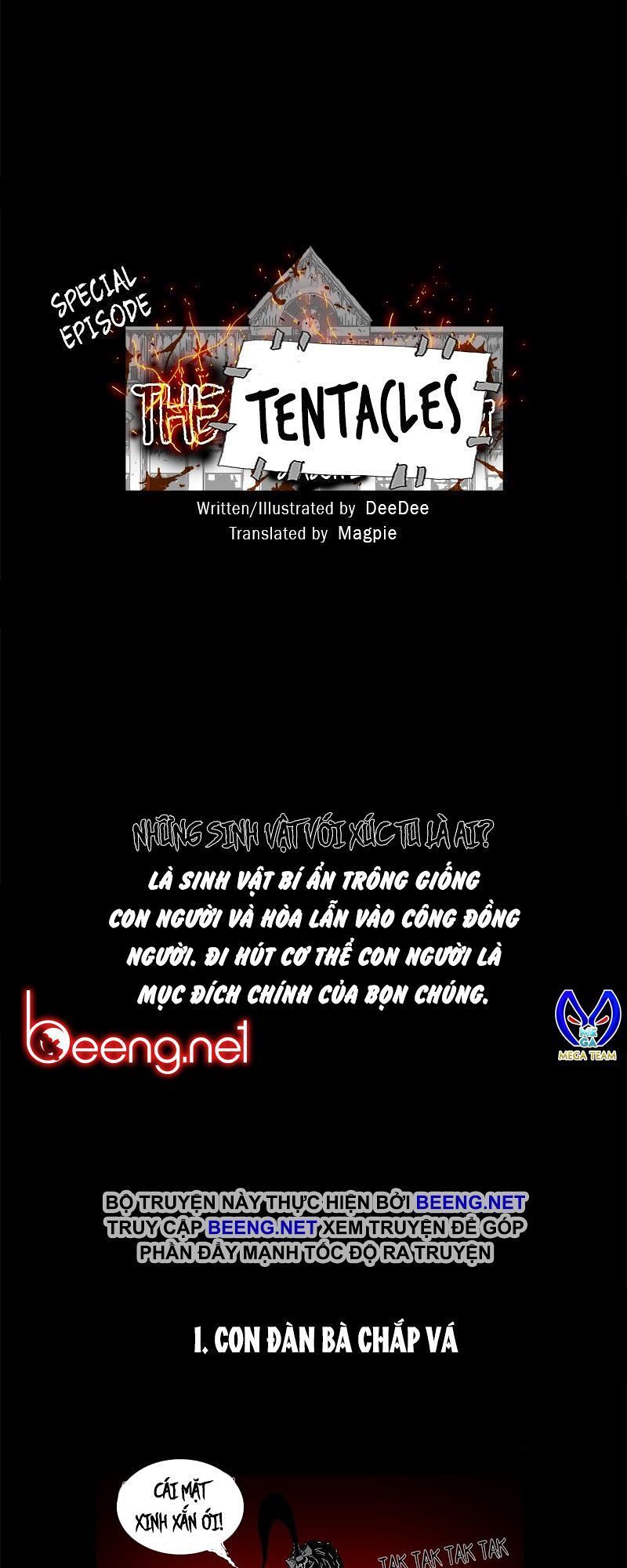The image features a black background and showcases a vertically oriented rectangular shape. At the top, there's a white piece of paper on a gray sign with some rings. Written prominently in a black, playful font on the paper is the title "The Tentacles." To the left of "The Tentacles," it's labeled as "special episode." This part is clear and easy to read. Below the title, there's additional text stating "Written and illustrated by Dee Dee and translated by Magpie." Underneath this text, there's more text written in an unidentified foreign language, possibly Asian. Further down, a comic strip-style speech bubble appears with more text in the same foreign language. On the left side, there is a reference to "beangele.net" in red, accompanied by an image that might resemble an angel with a heart, drawn in blue. The overall design implies that it may be an illustrated book or an online story with special episodes.